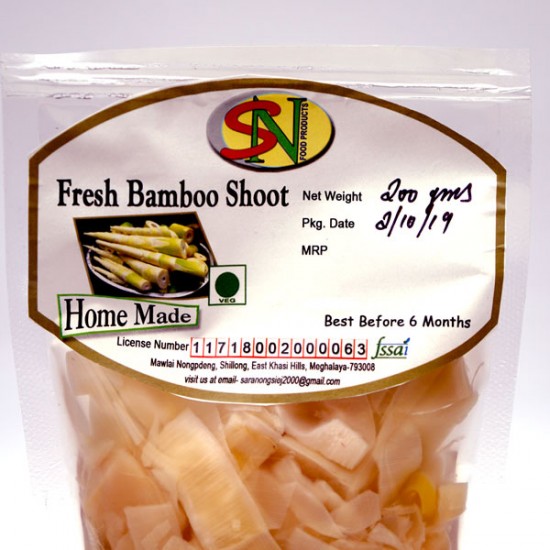This image displays a package of fresh bamboo shoots, encased in a clear plastic bag that reveals their light tan and white colors. The top half of the packaging prominently features a gold-bordered, white-filled label. Central to the label is the company logo: a stylized red "S" intertwining with a green "N" against a yellow oval backdrop. Above and below the logo, various details are printed. The label bears the words “food products” and “fresh bamboo shoot,” accompanied by images of bamboo and the word “homemade.” Specifics such as the net weight (200 grams), package date (February 10, 2019), and best before date (six months from packaging) are included, with some details handwritten. Additional text mentions the license number and geographic identifiers: Malay, Nong, Deng, Shillong, East Kalil Hills, and Magalia.